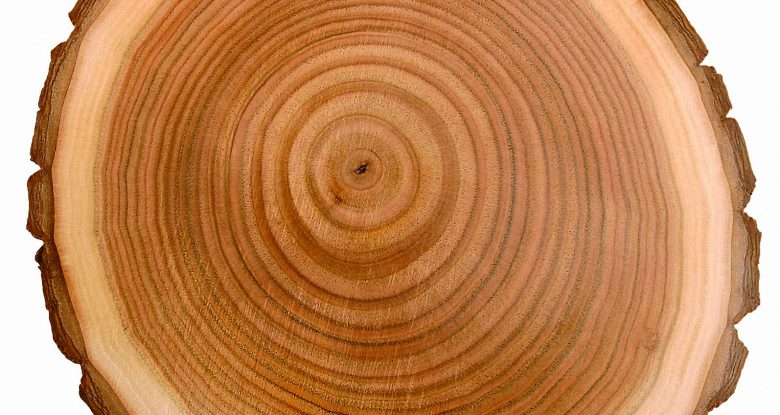The image is a horizontally aligned rectangular photograph showcasing a flat, round cutout from a log, likely intended as a decorative plate, platter, or platform. The wood slice reveals its natural rings and grains, starting with a very light tan color on the outer layer, becoming progressively darker towards the center, transitioning through medium brown to a very dark, almost black center. The outer edge still retains the rough, dark-colored bark, providing a textured frame around the smoother, circular inner rings. Set against a plain white background, the image focuses on the intricate, spiraled pattern of the tree's growth rings, emphasizing the contrast between the light outer rim and the dark center. The overall layout forms a rectangle, with the width being twice as long as the height, featuring visible portions of the bark along the top and bottom edges.